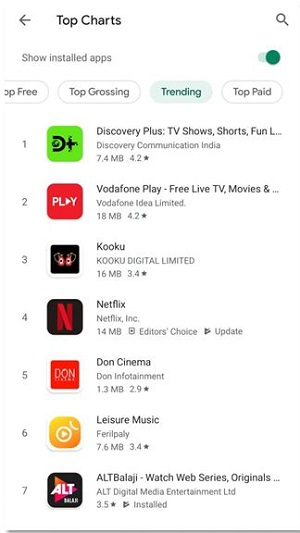The image appears to be a screenshot taken from a smartphone, showcasing a specific section of an app with a white background. At the top of the image, there is a left-pointing arrow icon, immediately followed by the text “Top Charts.” To the right of this text, there is a search icon. Below this bar, the text “Show Installed Apps” is visible, accompanied by a toggle switch that is turned on, indicated by its green color.

Further down, there is a row of tabs with the options: "Free," "Top Free," "Top Grossing," "Trending," and "Top Paid." The "Trending" tab is currently selected, and beneath it, a list of seven items is displayed, ranked accordingly.

1. **Discovery Plus**: The first item has a green square icon featuring the letters "D+." Its description reads, “Discovery Plus: TV Shows, Shorts, Fun, Discovery, Communication, India.” The app size is 7.4MB and it has a rating of 4.2 stars.

2. **Vodafone Play**: The second item has a red square icon with the word “Play.” It is described as “Vodafone Play: Free Live TV and Movies, Vodafone Idea Limited.” The app size is 18MB and it is rated 4.2 stars.

3. **Cuckoo Digital Limited**: The third item has a black square icon with eyes in it. The details state “Cuckoo Digital Limited.” The app size is 16MB and its rating is 2.4 stars.

4. **Netflix**: The fourth item features a black box with a red “N” for Netflix. It is described as “Netflix Incorporated.” The app size is 14MB and it is marked as "Editor's Choice" with an available update.

5. **Dawn Cinema**: The fifth item has a red square icon. Its description reads "Dawn Cinema: Dawn Entertainment.” The app size is 1.3MB and it has a rating of 2 stars.

6. **Leisure Music**: The sixth item shows a yellow circle icon with a play button. It is described as “Leisure Music.” The app size is 7.6MB and it has a 3.4-star rating.

7. **ALT Balaji**: The final item has a black box with "ALT" in white letters. The description reads "ALT Balaji: Watch, Web Series, Originals.” The app has a rating of 3.5 stars and is marked as "Installed."

This image effectively captures a detailed view of the trending apps as displayed in a mobile app store interface.